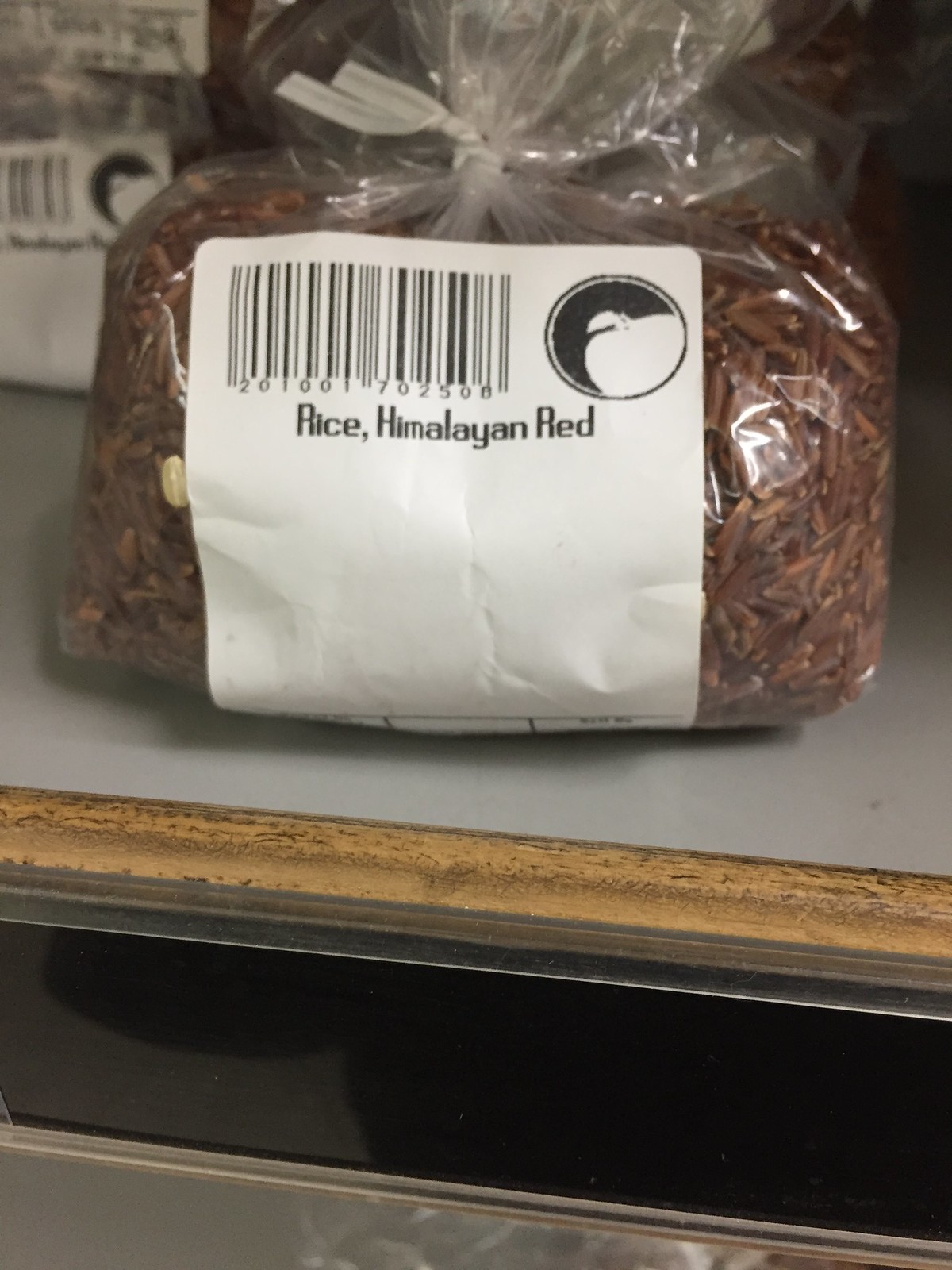The indoor color photograph prominently features a clear plastic bag containing dark brown rice, secured with a white twist tie. The bag is situated on a tan shelf with a brownish wooden edge. A white square label adorns the front of the bag, featuring a barcode in the upper left corner with the numbers 201-001 702508 below it. To the right of the barcode, there is a circular logo divided into black and white halves, reminiscent of a silhouetted bird's head or a white apple. Beneath the logo, in black text, are the words "rice, Himalayan red." Another similar bag of rice can be seen in the background on the upper left of the image. The bottom of the photograph displays a broad black rectangular area, slightly slanted, and a marbled dark gray triangular area.